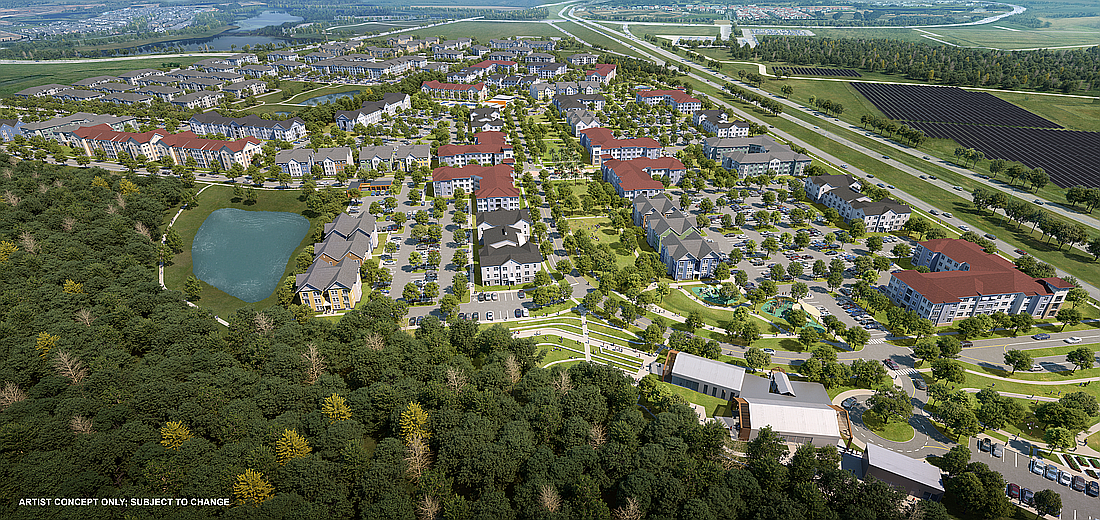The image presents an aerial view of a meticulously designed residential town characterized by its uniformity and cleanliness. The townscape is dominated by rows of cookie-cutter houses, predominantly white, with roofs in shades of red, gray, and dark brown. These residential areas are interspersed with abundant greenery, featuring trees of varied hues and densities. Towards the bottom left, a more wooded area extends significantly, providing a natural contrast to the structured environment. In the center-left section, a large, bluish-green lake offers a serene focal point amid the urban setting. The top right houses fields arranged in neat, darkly colored rows, potentially indicating agricultural use. Additional elements include a stretch of highway along the sides of the houses and some plains visible towards the right. A note at the bottom left corner states "artist concept only, subject to change," emphasizing the image’s conceptual nature. Overall, the scene reflects a modern, tidy, and well-planned community.